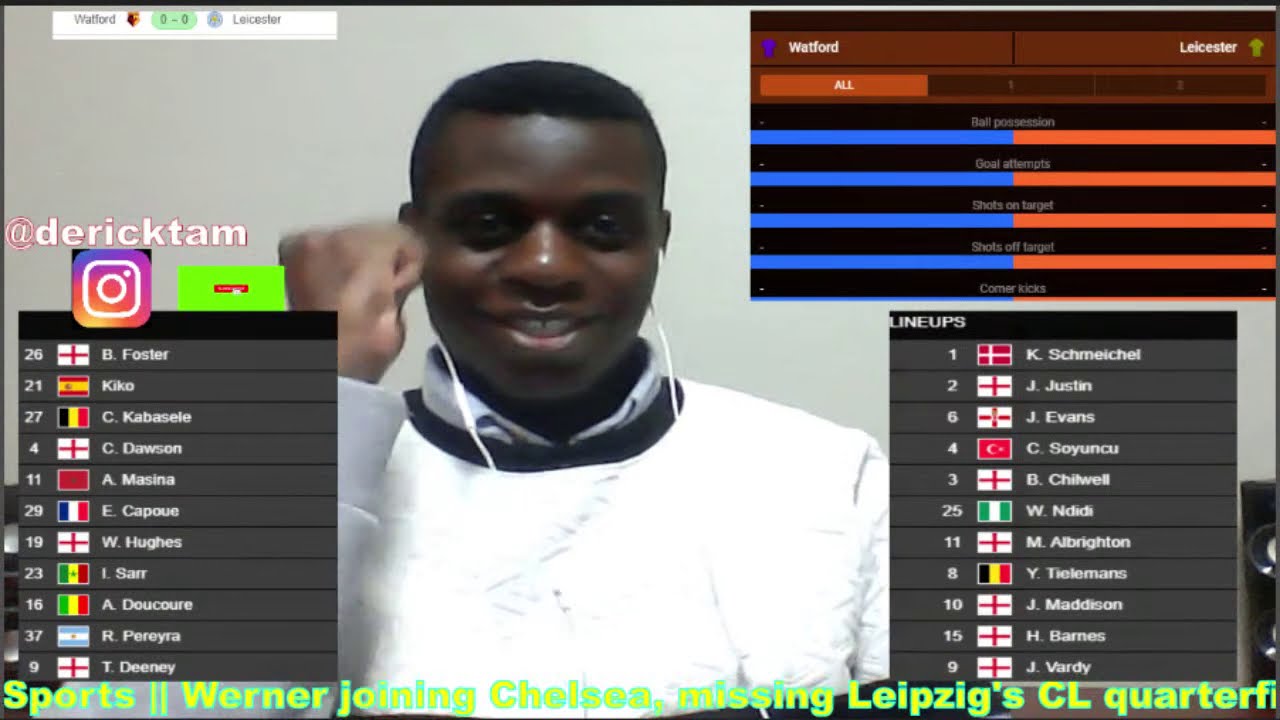The image depicts a televised sports broadcast displayed on a grayish background. At the center of the screen, an African-American man, donning a white sweater over a collared shirt, smiles warmly. He has short, black curly hair and appears to be wearing earbuds. Flanking him on both sides are statistical breakdowns. To the left, there are scores and country flags next to players' last names and initials. Similarly, on the right side, under a section labeled "Lineups," there are more flags and names. In the top right corner, a box displays team names—possibly "Westford" on the left and "Leicester" on the right—alongside four horizontal bars with blue and orange color-coding. At the bottom of the screen, a lime green ticker scrolls by with the word "Sports" and other ongoing updates, partially cut off on the right side.